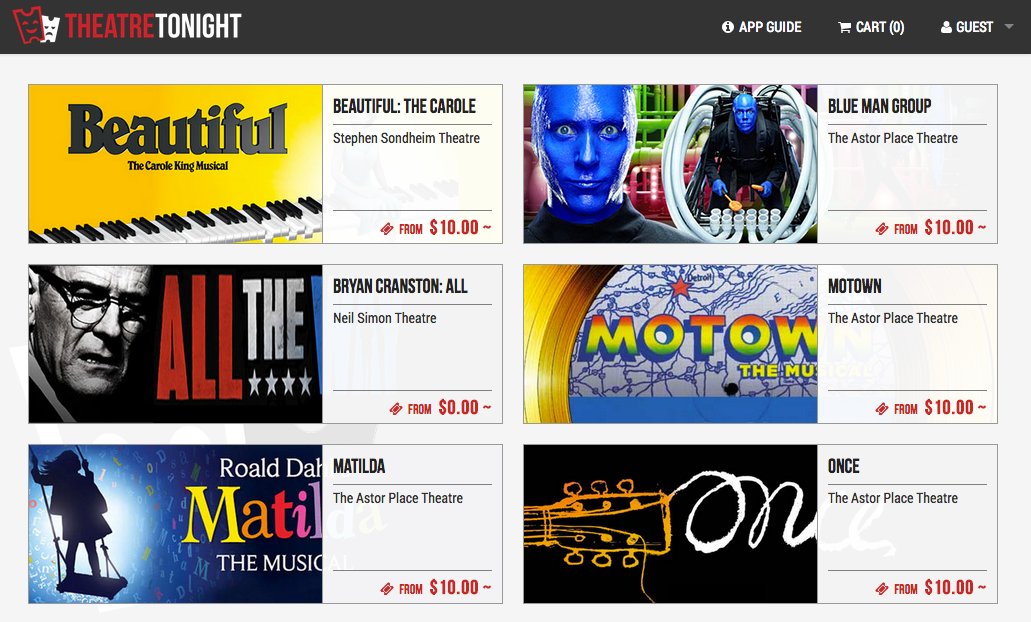The image appears to be a vibrant collage of various theater productions and promotional materials. Prominently featured are Red Tickets starting from $10 and multiple show advertisements. Highlights include "Beautiful: The Carole King Musical" and "Blue Man Group," noted for their distinctive blue-skinned performers with neon accents, associated with The Astro Plays Theater. Also mentioned are celebrity Brian Cranston and productions such as "Motown" and "Matilda." The latter is depicted with a blue background and a person standing on a swing. The image exudes a lively, colorful atmosphere with an assortment of text, graphics, and headshots interwoven throughout.